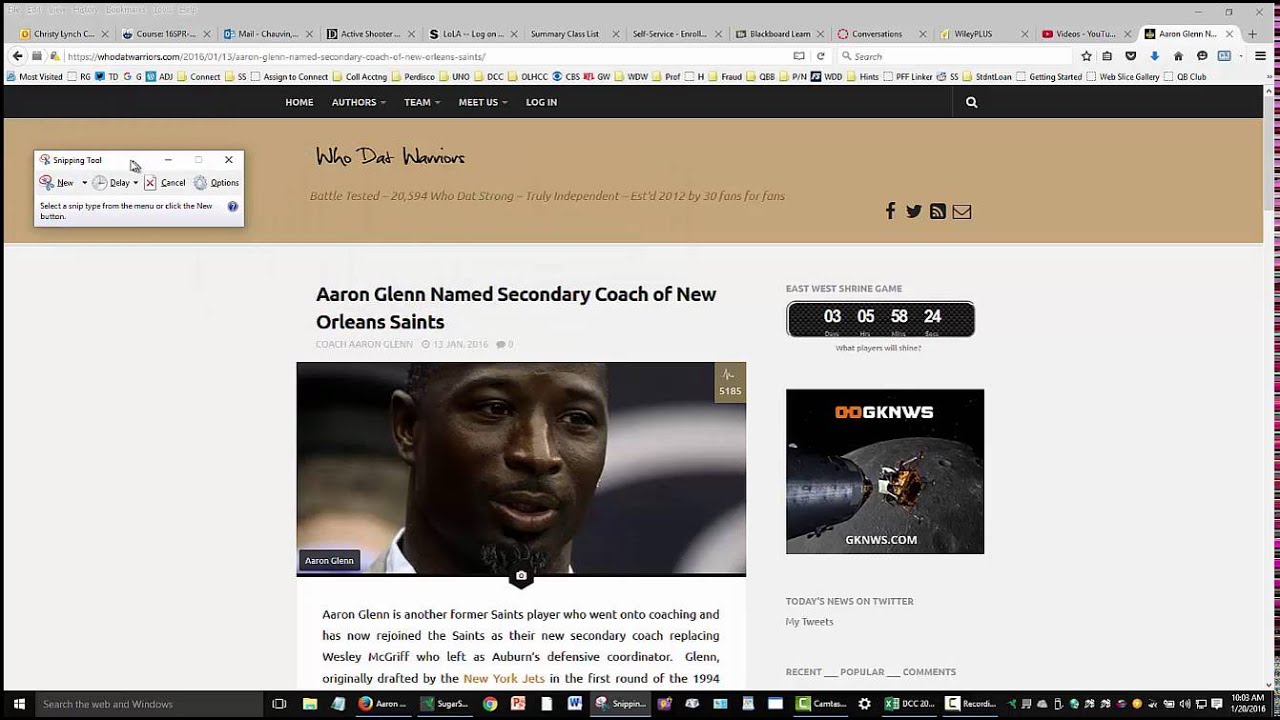The image showcases a horizontal screenshot of a webpage with detailed interface elements. At the top, a black icons bar includes labeled drop-down menus for "Home," "Authors," "Team," "Meet Us," and "Login." Below this bar is a thin beige banner strip presenting the webpage title, "Who Dat Warriors?" To the left of this strip is a pop-up box containing a tool menu, and to the right are various icons. 

The top header or banner of the page is light gray and features several open tabs, with the active tab positioned at the far right. Bookmark icons are also visible in this section, alongside the address and search bars.

The central section of the article prominently displays the headline, "Aaron Glenn Named Secondary Coach of New Orleans Saints," followed by a photograph of Aaron Glenn with associated black text. Adjacent to this content, on the right-hand side, is a countdown timer and an advertisement for GKNWS.

Finally, at the bottom of the screenshot lies the navigation bar, populated with numerous icons and open tabs. This bar integrates a search bar located on the left and the current time displayed at the bottom-right corner.